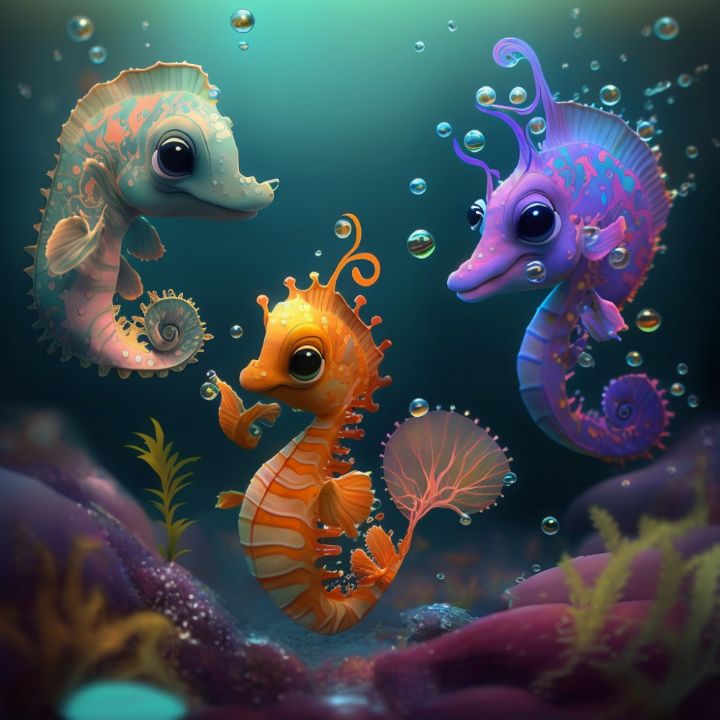A vibrant and colorful illustration, in an animated or airbrush style reminiscent of Pixar, depicts three seahorses floating in teal seawater filled with reflective bubbles. The center seahorse, predominantly bright orange with off-white banding and seaweed-like projections, looks to the left and has a large fan on its tail. To its upper left, a seahorse adorned in hues of peach, coral, and turquoise gazes to the right, seamlessly blending with its aquatic surroundings. The upper right seahorse stands out with its vivid purple, pink, and blue coloration, looking left with its tail fully curled. Below the trio, a blurred hint of a coral reef with various sea flora, including kelp and possibly starfish or anemone, adds depth to the scene. The artistic and detailed design, featuring exaggerated cartoonish eyes, suggests a playful and whimsical underwater world that could easily belong to a children's movie or advertisement.